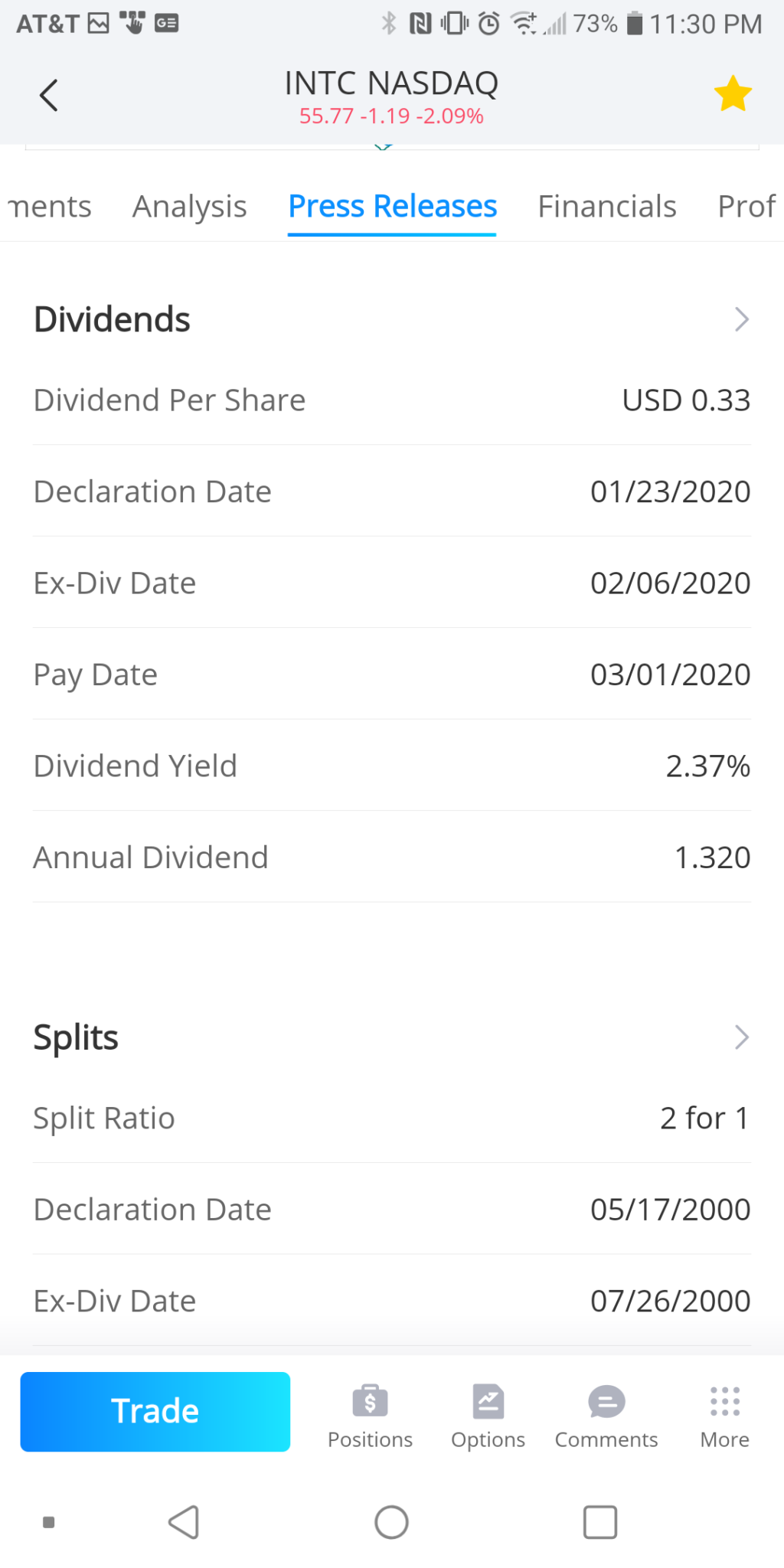At the top of the displayed page, there is a light blue header featuring several elements. On the left side, "AT&T 73%" is displayed, followed by "11:30 p.m." in the center. A left arrow is present before this text. To the right, "INTC NASDAQ" appears in black print, with stock information shown beside it: "55.77" in black, "-1.19" and "-2.09%" both in pink. There is a yellow star icon on the far right.

The body of the page has a white background with various sections labeled in gray print. The "Mints Analysis and Press Releases" section is highlighted in blue, accompanied by a blue underline. 

Further down, the "Financials" and "Pro" sections are present, followed by subsections labeled "Dividends," which details: 
- Dividend Per Share
- Declaration Date
- Ex-Div Date
- Pay Date
- Dividend Yield
- Annual Dividend

This section features corresponding dates and amounts for user reference.

Following this, the "Splits" section provides:
- Split Ratio: 2-for-1
- Declaration Date: 05/17/2000
- Ex-Div Date: 07/26/2000

There is a blue button with a gradient effect, labeled "Trade," featuring white text inside it.

Below are additional sections such as "Positions," "Options," "Comments," and "More."

At the very bottom, there are graphical symbols including a black dot, and a white triangle, circle, and box.